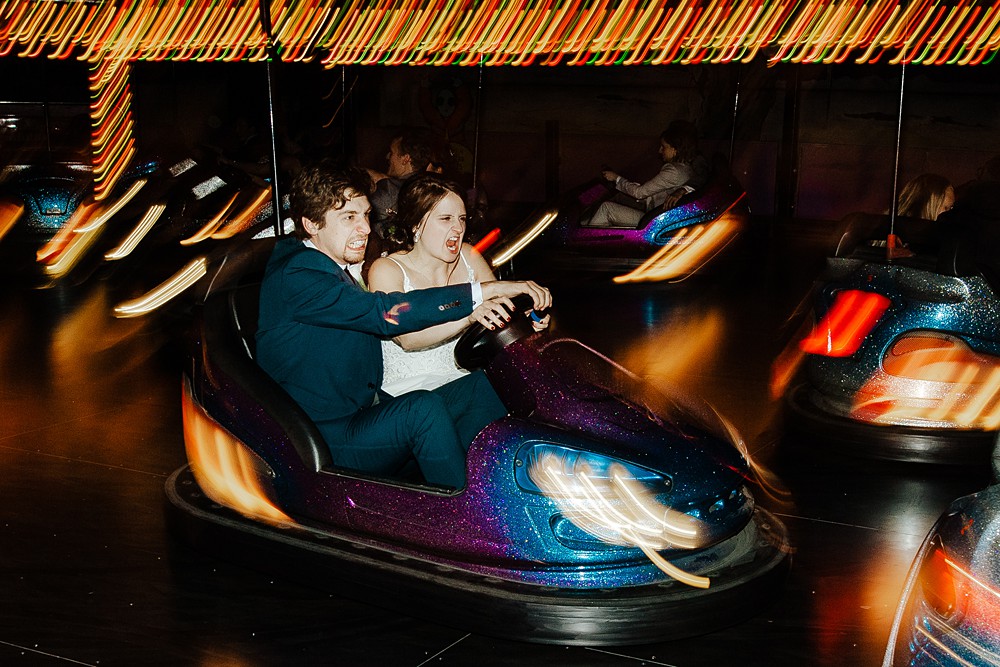The photograph captures an exhilarating bumper car exhibit inside a dimly lit venue. In the foreground, a young couple is intensely engaged in the thrill of driving an iridescent purple and bluish glittery bumper car, adorned with motion-blurred lights on both the front and back. Their faces, adorned with grimaces that could be mistaken for anger, actually reflect their excitement and aggressive determination to collide with other riders, which is the spirited objective of the game. The young man, recognizable by his goatee and blue suit that reflects the multi-colored lights around, grips the steering wheel with his right hand, while the young woman in a white sleeveless shirt mirrors his focused expression and also holds the wheel. The scene around them is dynamic, with other single riders visible in their bumper cars, all navigating towards inevitable impacts. The backdrop is notably dark, punctuated by vibrant light trails from the fast-moving cars, creating a lively and somewhat blurred effect, adding to the motion and energy of the moment. This snapshot, despite its slight overexposure, vividly captures the fun and intensity of a possible date night at the bumper car arena.